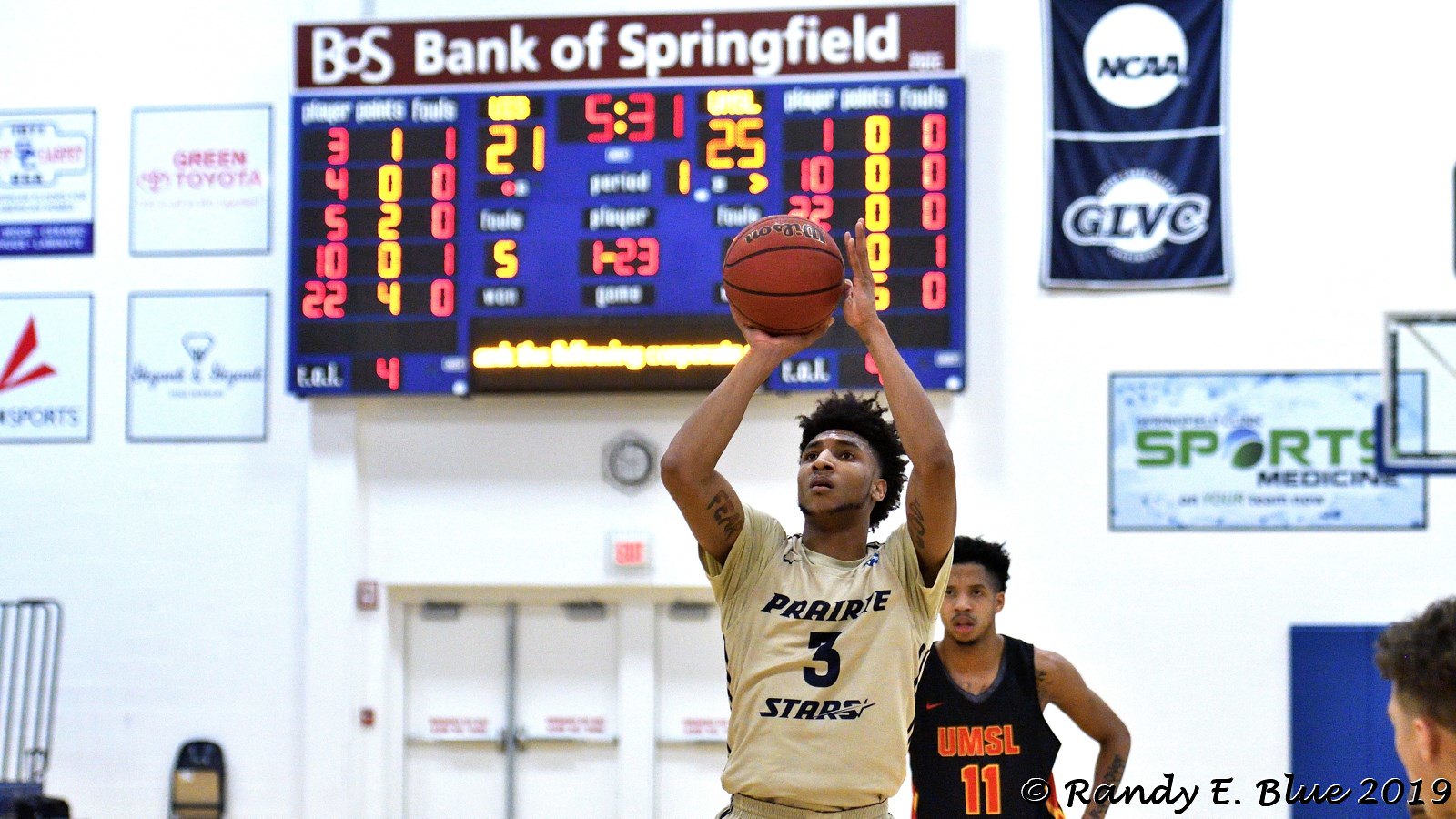This professional photograph captures an intense moment in a basketball game. At the forefront, a player wearing a white jersey with the number 3 is poised to take a shot, lifting the basketball above his head. His jersey reads "Prairie Stars" across the front in black letters. Visible on his left bicep is a tattoo that spells "F-E-A-R," while another tattoo is partially visible on his right bicep. Standing behind him, an opposing player in a black jersey with red lettering is marked by the number 11 and the team name "UMSL."

In the background, a large electronic scoreboard sponsored by the Bank of Springfield (BOS) prominently displays the score of 21 to 25 in orange digits, with a timer reading 5:31 in red. Additional details from the scoreboard include player points and fouls. The wall behind them is peppered with various sponsor logos, emergency exit doors, and flags including the NCAA and GIVC. A sports medicine banner is also visible, contributing to the collage of sponsorship. At the bottom of the image is a copyright notice from Randy E. Blue dated 2019.